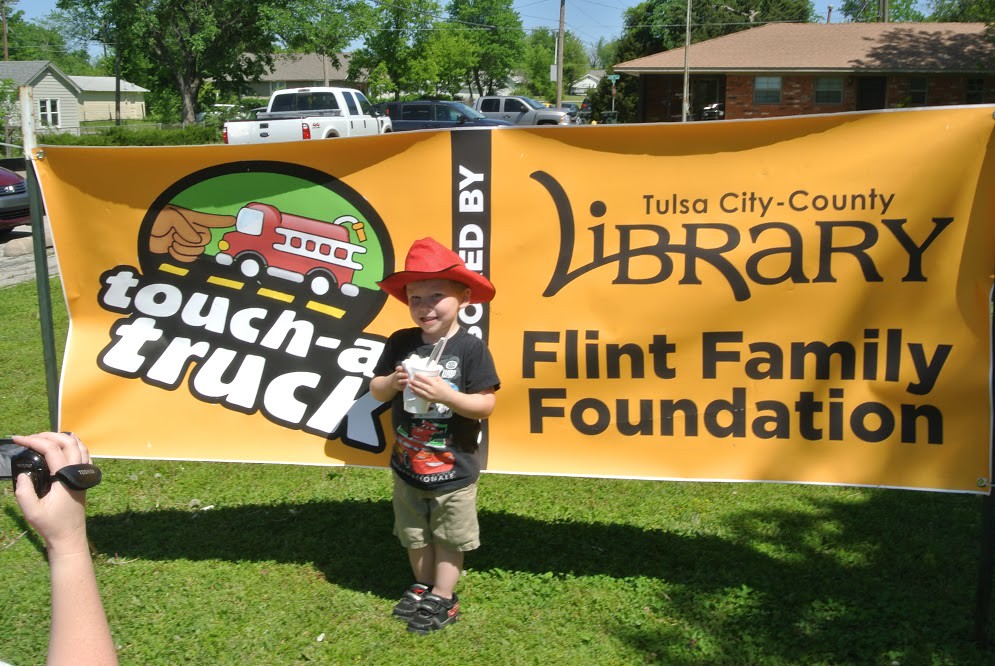In this vibrant outdoor photo, a cheerful young boy, around five years old, stands centered on a grassy area. He is clad in a black graphic T-shirt featuring characters from the movie "Cars," tan khaki shorts, and black sneakers. The boy's playful appearance is accentuated by a red firefighter's hat, and he holds a cup with a spoon sticking out, which presumably contains ice cream. Behind him, a tall, orange banner staked to the ground proudly displays, "Touch a Truck," accompanied by a colorful drawing of a large hand touching a cartoon fire truck on the road. Further text on the banner reads, "Tulsa City-County Library Flint Family Foundation." The scene captures a sunny, beautiful day, likely in a quaint town setting hinted by visible buildings, cars, and streets in the background. A hand is visible in the bottom right corner, capturing the moment on a handheld camera, adding a personal touch to the lively and warm atmosphere.